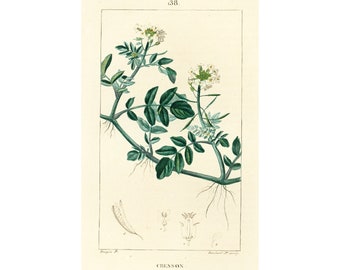This image captures a vintage, botanical illustration that resembles a poster or a page from an old book, characterized by its off-white or tan paper that has aged to a slightly yellowed tone. The artwork showcases a green plant with rich, oval-shaped leaves, hand-drawn or hand-painted in a classic vintage art style. Distinguishing features of the plant include cylindrical tufts, resembling dandelions, with delicate white puffs attached to a green center. Several thin roots can be seen extending from the plant, seemingly suspended in mid-air at various points. The composition is framed by a thin black border that stretches from the left to the right side of the paper. Small, faded brown text appears both at the top and the bottom of the page, likely serving as a description, though it is difficult to decipher. Overall, the piece has an antique feel, emphasized by the paper's aged appearance and the detailed botanical rendering.